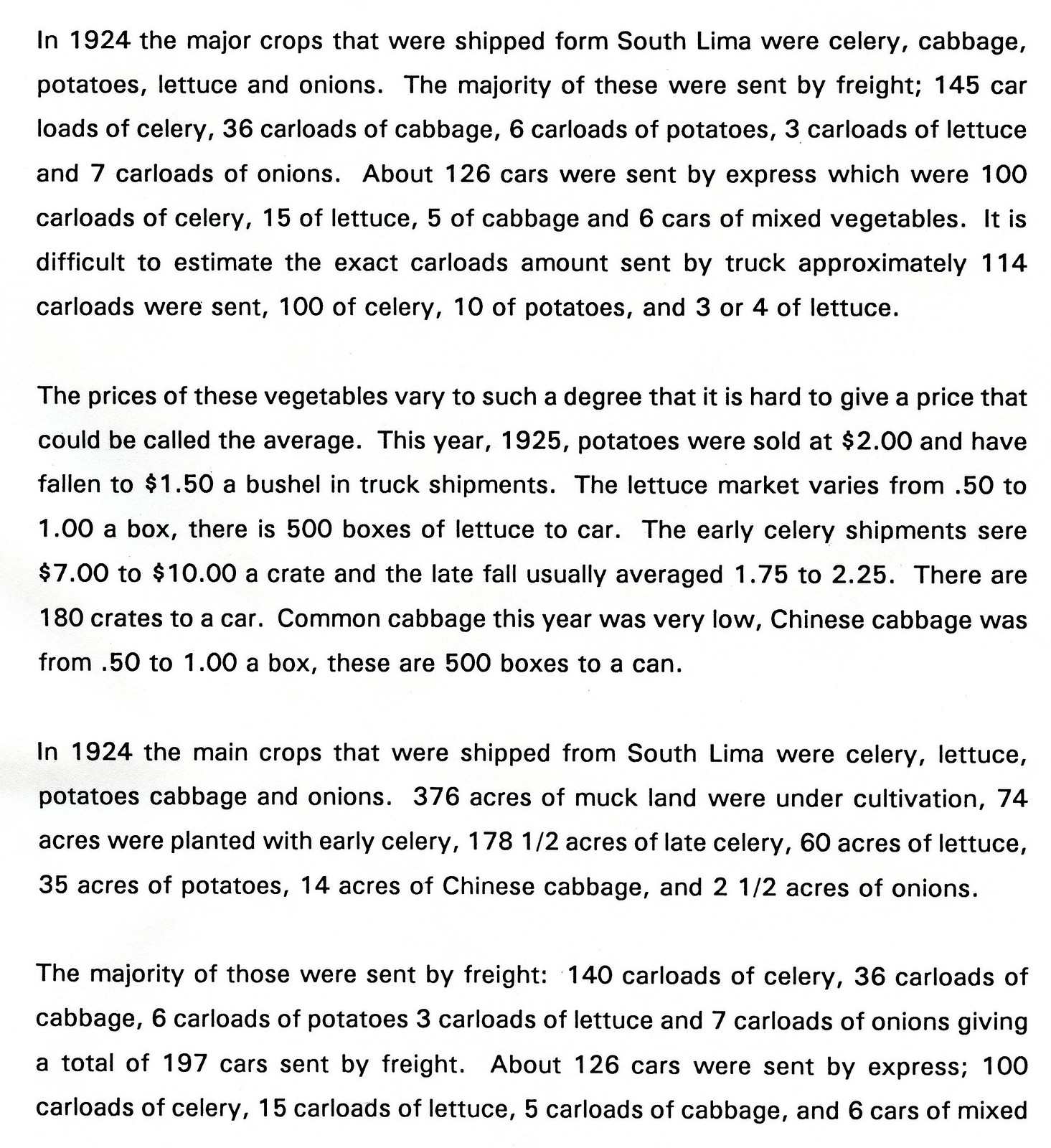The image presents a detailed black text on a white background, with four paragraphs focusing on the agricultural outputs of South Lima in 1924. The main crops shipped from South Lima in that year included celery, cabbage, potatoes, lettuce, and onions. Notably, freight was the primary method of transportation, with 140 carloads of celery, 36 carloads of cabbage, 6 carloads of potatoes, 3 carloads of lettuce, and 7 carloads of onions, totaling 192 carloads sent by freight. Additionally, about 126 carloads were sent by express, comprising 100 carloads of celery, 15 of lettuce, 5 of cabbage, and 6 carloads of mixed vegetables. Truck transportation accounted for approximately 114 carloads, including 100 carloads of celery, 10 of potatoes, and 3 or 4 of lettuce. The text emphasizes the variability in vegetable prices, making it challenging to ascertain an average price. For example, in 1925, potato prices fell from $2 to $1.50 per bushel. Lettuce prices ranged from $0.50 to $1 per box, while early celery shipments fetched between $7 and $10 per crate, decreasing to $1.75 to $2.25 for late fall shipments. Cabbage prices fluctuated significantly, with common cabbage being particularly low and Chinese cabbage costing $0.50 to $1 per box.